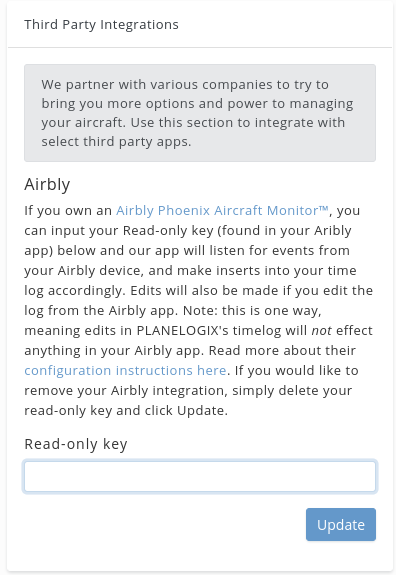This image features a clean white background with a thin gray border running along the right side. In the top left corner, the text "Third Party Integrations" is prominently displayed in black. Just beneath this text, there's a thin gray line followed by a light blue rectangle containing four lines of black text. The text within the rectangle reads: 

"We partner with various companies to try to bring you more options and power to managing your aircraft. Use this section to integrate with select third party apps."

Below this, the white background continues on the left side with the bold black text "AirBLY" clearly standing out. The subsequent section begins with "If you own" in black text, followed by the blue trademarked phrase "Arably Phoenix Aircraft Monitor™." It continues:

- "you can input your read-only key found in your Arably app.
- Our app will listen for events from your Arably device and make entries into your time log accordingly. 
- This will be made if you edit the log from the Arably app. 
- Note: This is one-way, meaning edits in Jaunt Planer’s time log will not affect anything in your Arably app. Read more about their configuration instructions here."

Following this section, additional black text outlines the removal process for the integration:

"If you like to remove your Arably integration, simply delete your read-only key and click update."

Towards the bottom left of the image, the text "Read-Only Key" is displayed above a long white rectangle outlined in light blue. In the bottom right corner, a noticeable blue tab with white text reads "Update."